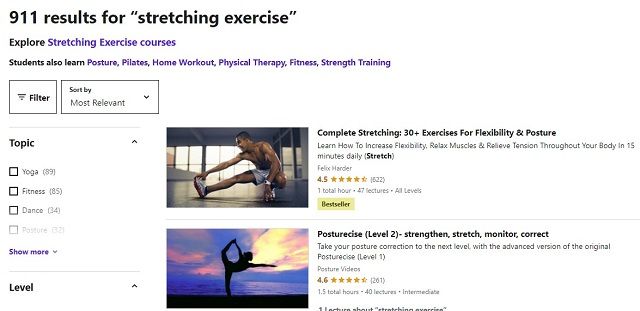The image is a horizontal-oriented screenshot of a webpage, featuring a clean, white background without a border. In the upper left-hand corner, "911 results for stretching exercise" is prominently displayed, followed by the suggestion to "Explore stretching exercise courses." Additional topics such as posture, Pilates, home workout, physical therapy, fitness, and strength training are mentioned for further learning. Below these, two small buttons outlined in a thin gray line read "Filter" and "Sort by," indicating that the results are currently sorted by "Most Relevant."

On the left side of the main image, a sidebar with "Topics" and "Level" categories is visible, both equipped with small arrows for scrolling through options. To the right, the main content area features two photographs. The top photograph depicts a muscular man kneeling down on the floor, stretching out his right calf, with the caption "Complete Stretching: 30+ Exercises for Flexibility and Posture." This course has a rating of 4.5 stars and is marked as a "Bestseller." 

Below this, another image shows a silhouette of a person performing a yoga pose against a sunset with purple and yellow hues. The caption reads "Posture Size Level Two: Strengthen, Stretch, Monitor, and Correct." This course also includes a brief description underneath and boasts a rating of 4.6 stars.